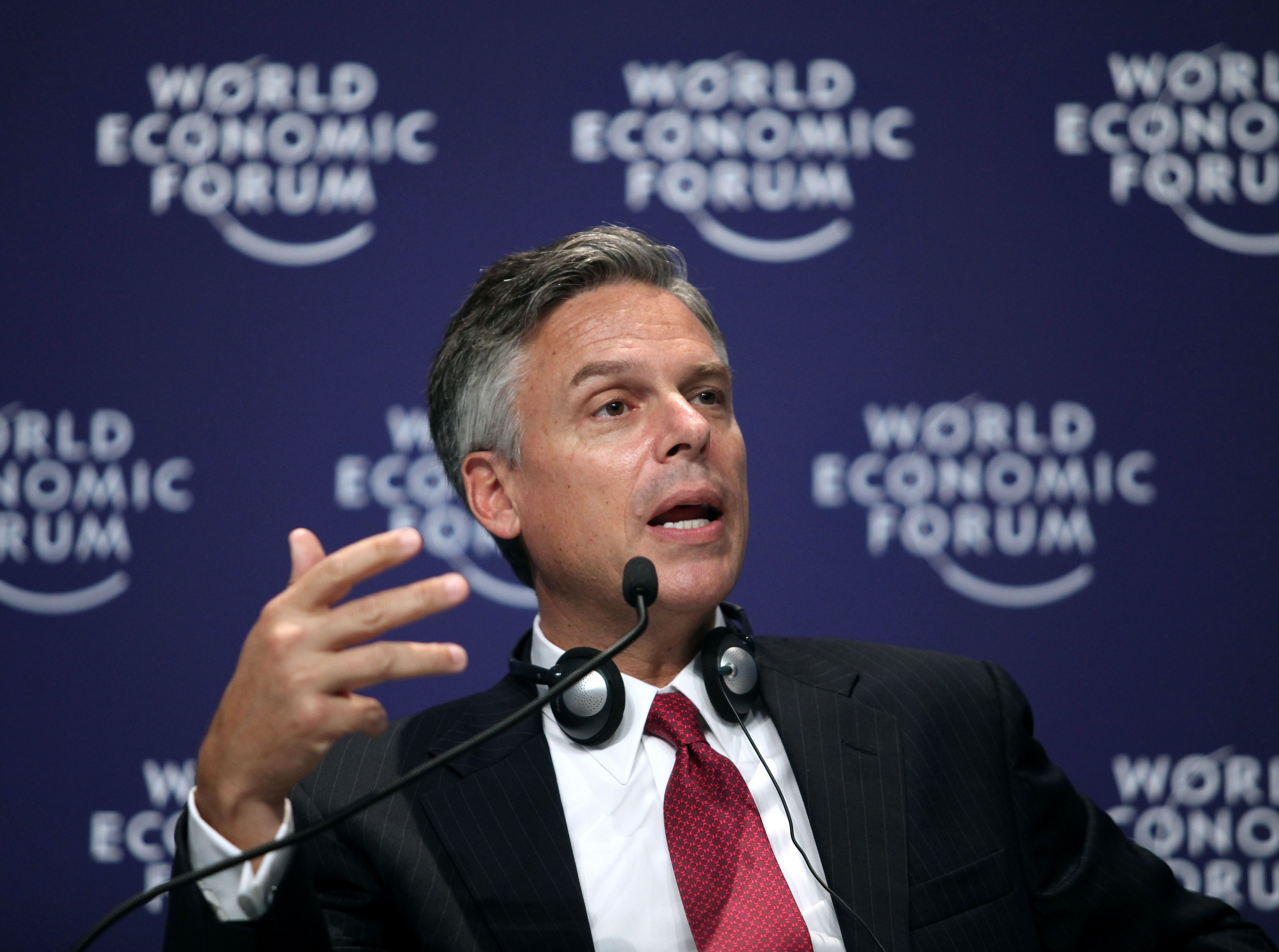The image depicts a man positioned centrally, either standing or sitting, against a blue backdrop adorned with the repeating text "World Economic Forum" in white. The man, captured from below the chest upward, is engaged in speaking into a thin microphone that extends from the bottom left of the image towards the center. He has short hair that is brown on top and gray at the sideburns. His mouth is open, indicative of active speech, and his right hand is raised in front of his shoulder. He is dressed in a dark suit jacket, a white shirt, and a distinctive pink tie with black dots. Around his neck, he appears to be wearing headphones. The image is likely taken indoors, possibly at a press conference or similar event, featuring a color palette that includes purple, white, black, gray, tan, pink, and red. While the man is sharply in focus, the background text is slightly blurred but still legible.